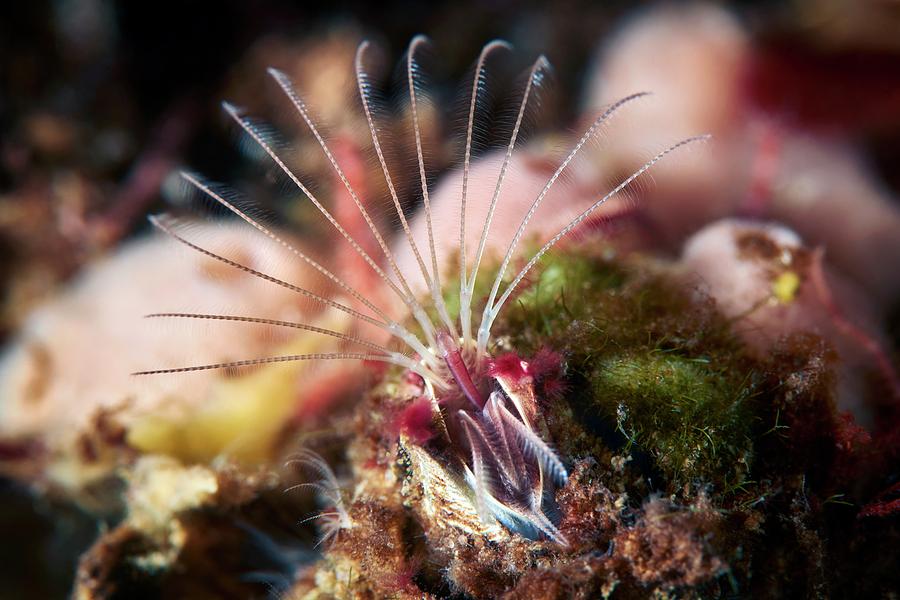In this underwater photograph, we are presented with an extreme close-up of a fascinating sessile creature residing among a vibrant coral reef. The central figure in the image is a uniquely intricate organism, featuring a broad, feathery fan-like structure emerging from a base decorated with petal-like appendages in hues of blue and magenta. The fan's individual feathers are fine and delicate, with a central striped fiber leading to tips adorned with exceedingly fine, short filaments that appear to emit a faint blue glow.

From the creature's mouth, barbed tendrils extend outward, adding to its alien and captivating appearance. Surrounding the base, a variety of plant life can be observed, including a greenish moss and a brownish type of moss, along with other grass and moss-like vegetation. The blurred background hints at the complexity of the underwater environment, which includes structural coral reefs, enhancing the composition with their subtle yet essential presence. The overall scene is a detailed tableau of life in the depths, showcasing the intricate beauty and biodiversity of the ocean.